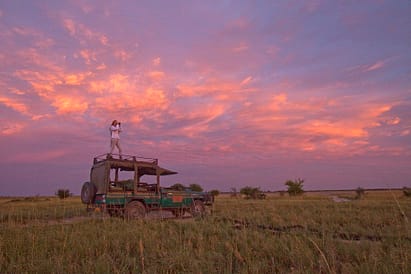In a sweeping, desolate grassland that stretches out into the horizon under a striking twilight sky tinged with oranges, pinks, and purples, an older, green off-road expedition vehicle, reminiscent of a classic Land Rover, stands prominently. The landscape, which recalls the vastness of African or Australian wilderness, is dotted with sporadic small shrubs amidst the dry, green fields. Atop the vehicle's open-air canopy, a woman dressed in a white long-sleeved shirt and cream-colored pants surveys the scene through binoculars, seemingly capturing a photograph. The unique hues of the sky, interspersed with orange clouds, and the serene aura of the natural setting accentuate the adventurous spirit of the scene.